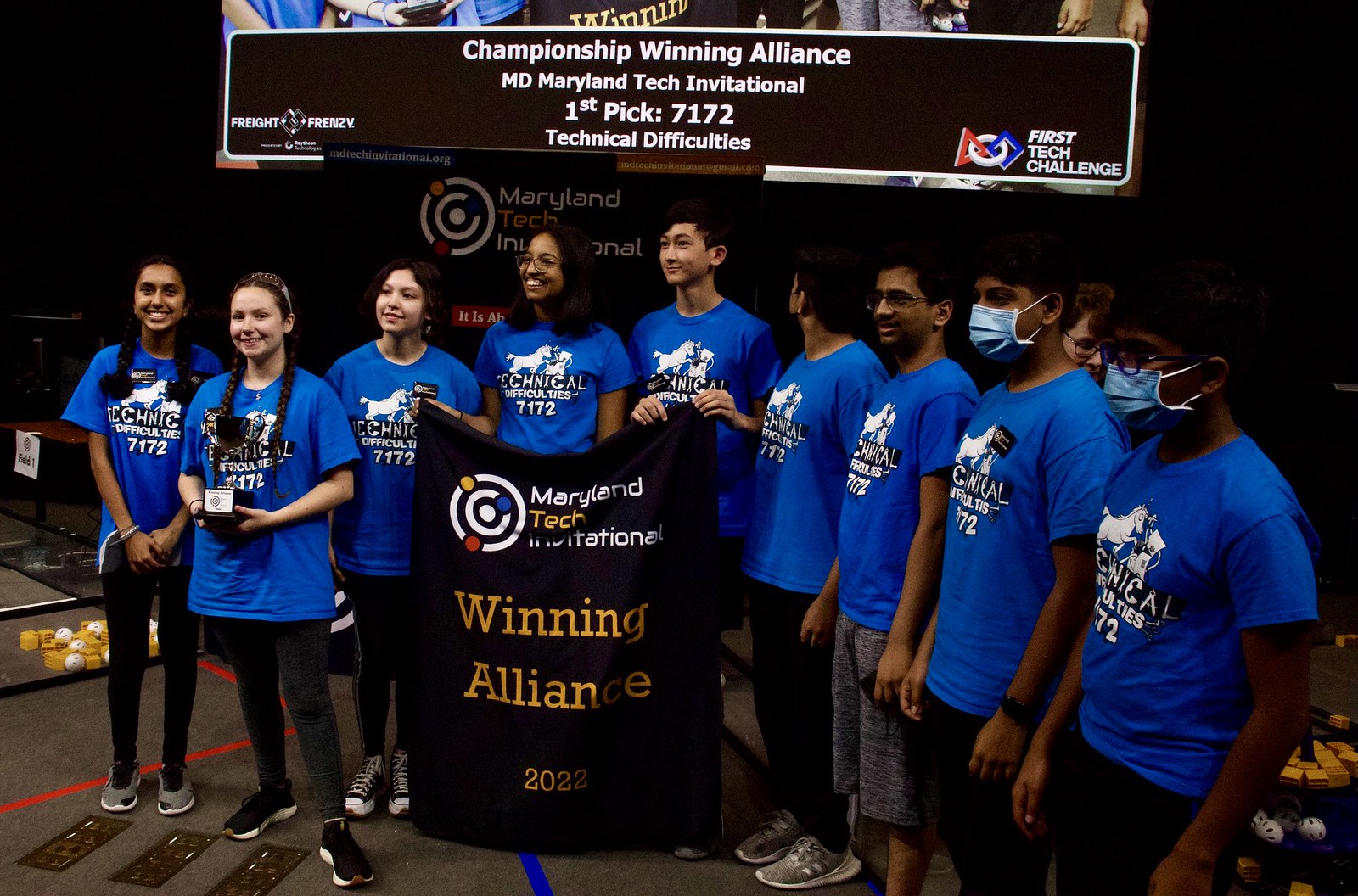This photograph captures a jubilant group of high school students, approximately ten, arranged in a semi-circle and proudly displaying matching blue t-shirts with a white and black logo. The teens, a diverse mix of predominantly Asian and Indian backgrounds, include four girls and five boys, all smiling and visibly excited, with two of them wearing masks. 

At the center of the group, two members hold a prominent black banner that reads "Maryland Tech Invitational Winning Alliance 2023" in bold yellow text. Behind them, an overhead sign reinforces their victory, declaring "Championship Winning Alliance Maryland Tech Invitational First Pick 7172 Technical Difficulties," and annotating their affiliation with "First Tech Challenge."

Adding to the vibrant scene, the background partially obscures another sign, with legible portions stating "Maryland Tech," next to a logo. Small yellow squares and round balls are scattered at the bottom left of the image, with more of these objects visible on a table to the lower right, suggesting a competitive tech setting.